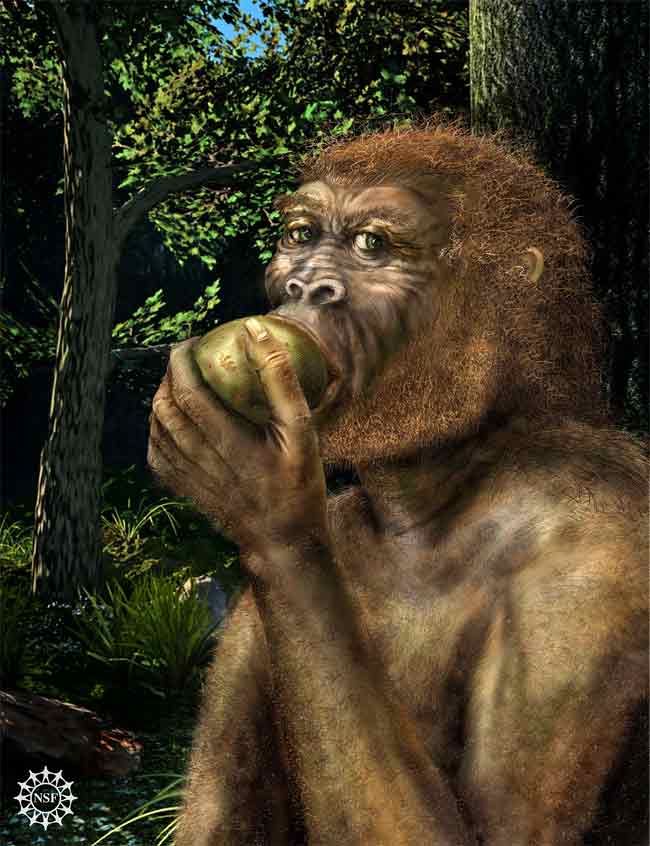This image features a semi-realistic, slightly stylized depiction of a monkey, characterized by its light brown head hair and darker brown facial and body hair, which is sparse in coverage. The monkey is engaged in eating a green fruit, likely an apple, which it holds in its left hand while its mouth is around it. The scene is set against a forest backdrop, showcasing various trees with lush green foliage. On the left side, a prominent tree extends upwards with a branch halfway up adorned with leaves, and at its base are rocks, grass, and some weeds. Another tall tree occupies the right side, towering with visible greenery at the top. The monkey, positioned about two-thirds down on the right, is slightly turned left, facing the front with its eyes directed toward the camera. There is a patch of blue sky visible behind the trees. In the lower left corner of the image, a white logo resembling a ship's steering wheel with spokes shaped like people holding hands bears the initials "NSF."